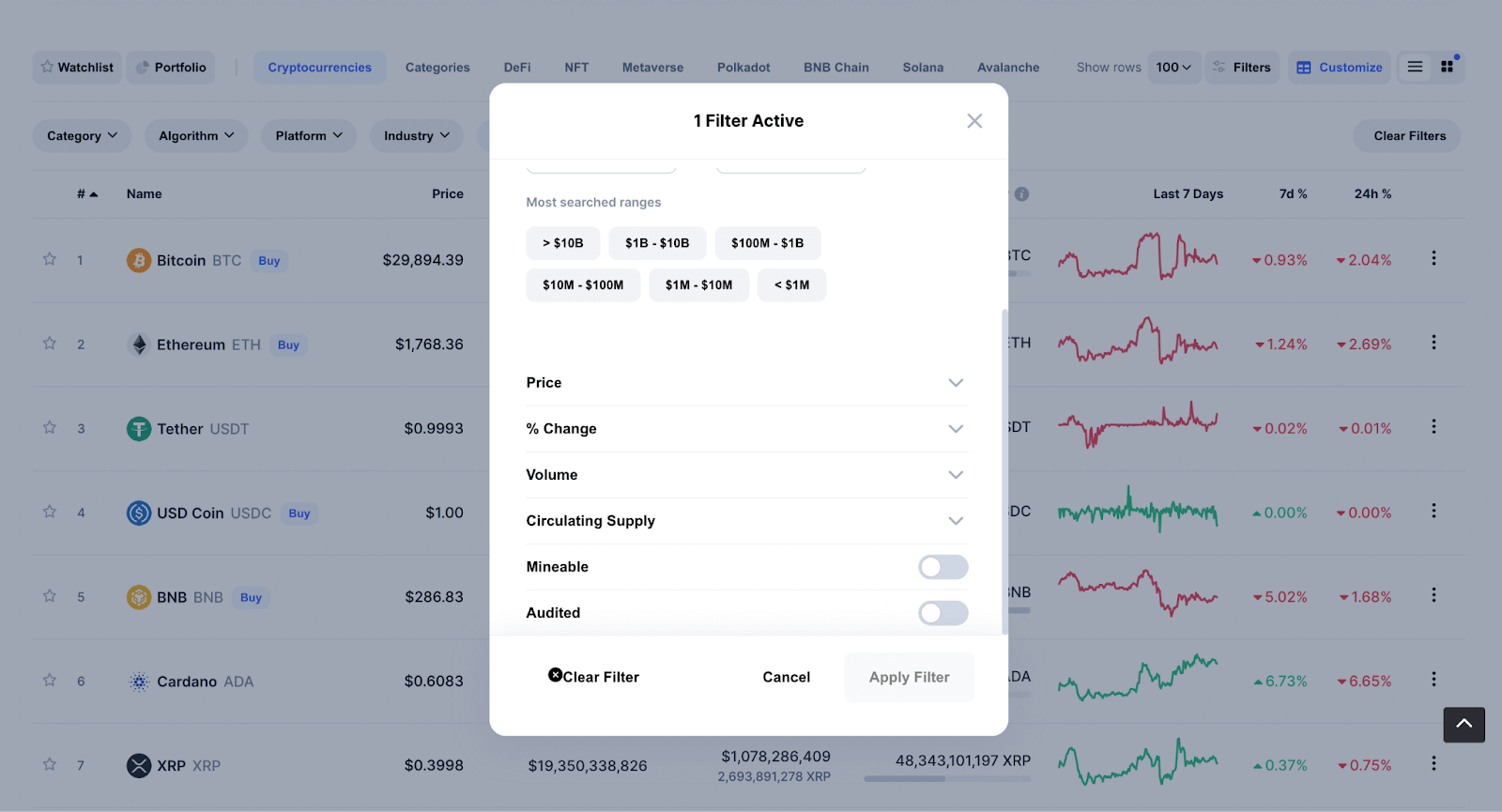The web page displayed appears to be related to the financial market, specifically focusing on stocks or cryptocurrencies. In the background, the main screen features detailed information on various cryptocurrencies, including Bitcoin, Ethereum, Tether, USD Coin, Binance Coin (B&B), Cardano, and XRP. Each cryptocurrency is listed with its corresponding price: Bitcoin is $29,894.39, Ethereum is $1,768.36, Tether is $0.9993, USD Coin is $1.00, Binance Coin is $286.93, Cardano is $0.60, and XRP is $0.39.

Overlaying the main screen is a pop-up window which states "One filter active." This pop-up provides various sorting and filtering options, such as "most search engine ranges" along with dollar amounts. It displays metrics including price, percent change, volume, circulating supply, amendable and audited statuses, as well as options to "clear filter" and "cancel."

To the right of the main screen, there is a bar graph illustrating the price movement and trends for the past seven days, similar to stock market charts showing fluctuations over time.